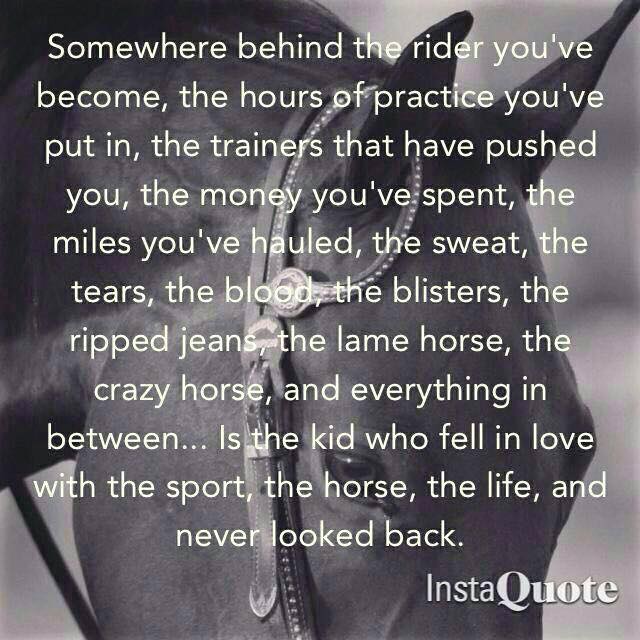The image is a close-up, black-and-white photograph of a horse’s head, showing its eyes, ears, part of its neck, and shoulders. The horse is looking to the right and wearing a bridle adorned with rhinestones. The photo, formatted as a square graphic ideal for social media platforms like Facebook or Instagram, features prominent white text overlaying the image. The text reads: "Somewhere behind the rider you've become, the hours of practice you've put in, the trainers that have pushed you, the money you've spent, the miles you've hauled, the sweat, the tears, the blood, the blisters, the ripped jeans, the lame horse, the crazy horse, and everything in between is the kid who fell in love with the sport, the horse, the life, and never looked back." In the bottom right corner, the logo for InstaQuote is visible.